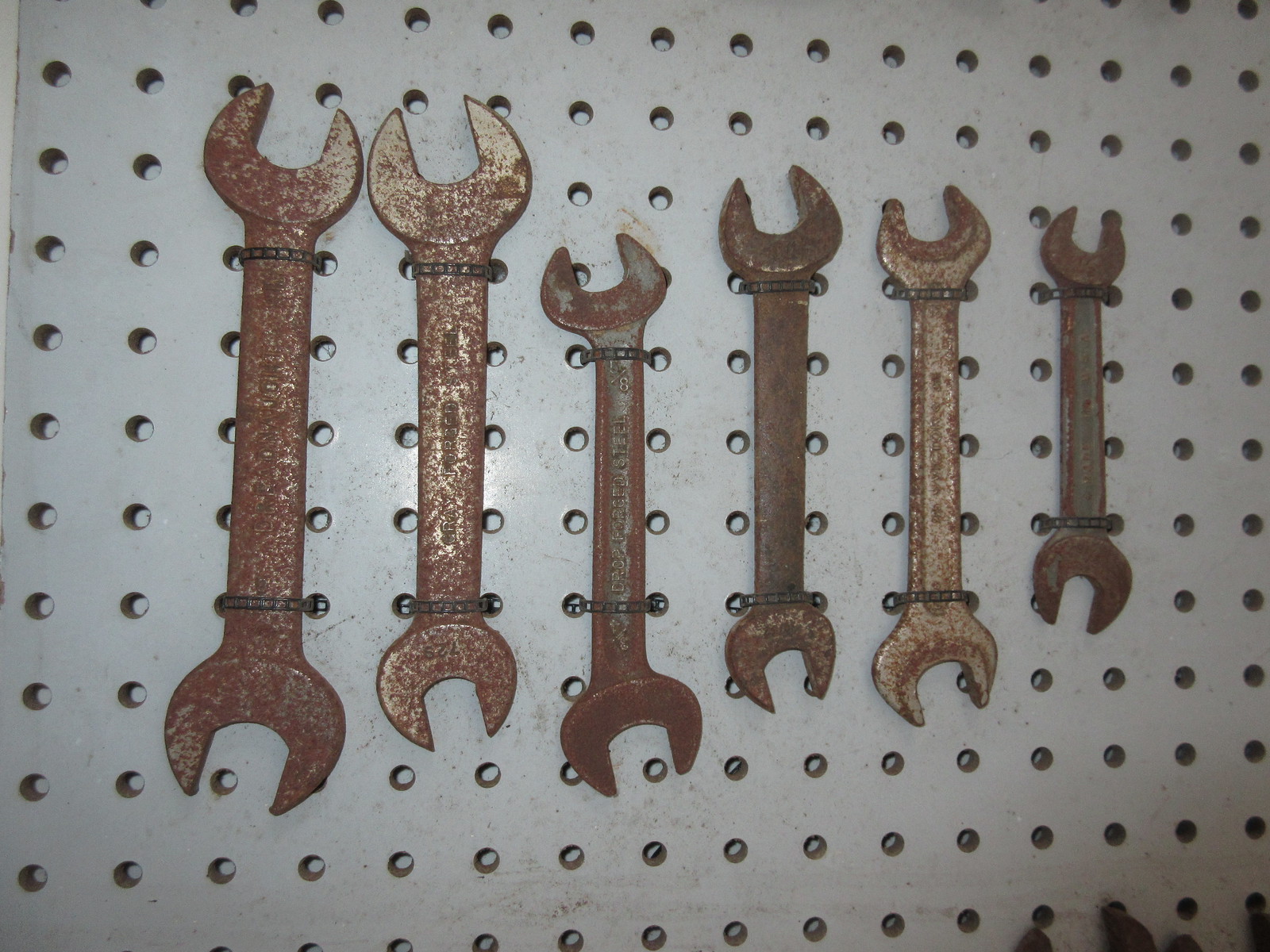The image depicts a section of a tool shed with a white pegboard mounted on the wall. The pegboard, characterized by evenly spaced holes, is set up in a 10-row by 17-column grid pattern, precisely one inch apart from each other. Affixed to this pegboard, in the approximate middle to top area, are six rusted wrenches of varying sizes, meticulously organized from the largest on the left to the smallest on the right. Ranging from heavily rusted brown to patches where the underlying silver metal is visible, these wrenches are firmly secured with twist ties threaded through the pegboard holes. All wrenches show signs of extensive use and are arranged in descending size order: the two largest wrenches lie on the left, followed by two medium-sized ones, and finally the two smallest on the right. Some text, likely indicating the size and brand, is partially visible on the wrenches despite the rust. Towards the bottom right of the image, there appears to be a pair of gloves hanging, suggesting the utilitarian nature of the space. This detailed photograph seems to capture an organized yet worn collection of tools, possibly for documentation or sales purposes.